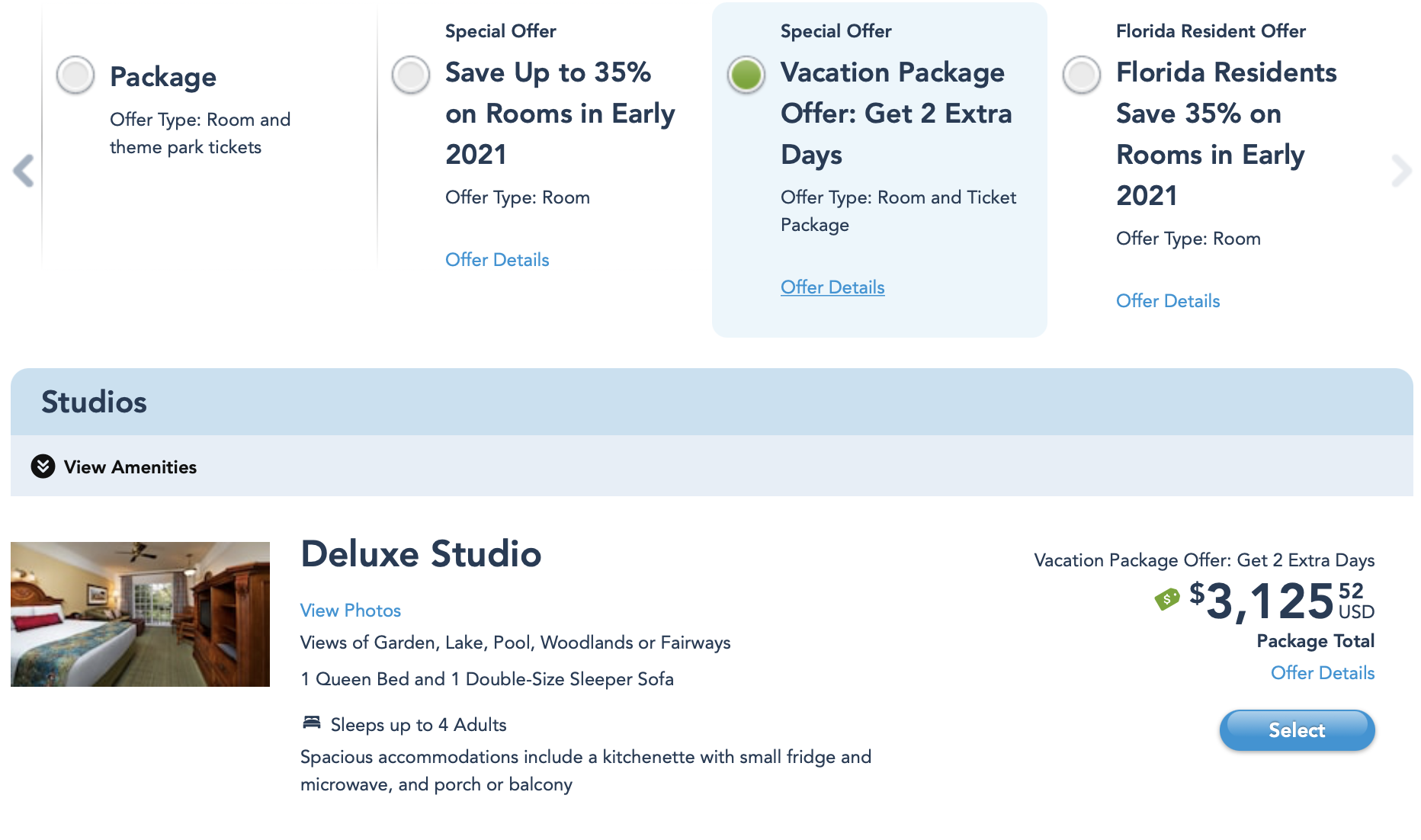Screenshot of a vacation rental website displaying various apartment options and special offers. At the top of the webpage, there are four promotional tabs: "Package," "Special Offer," "Special Offer," and "Florida Resident Offer." The "Vacation Package Offer" is selected, which provides an additional two days with a room and ticket package. A clickable "Offer Details" dialogue is available under three of the options, excluding the "Package" tab.

Below the promotional tabs, there is a section labeled "Studios" for studio apartment types, accompanied by a "View Amenities" link. The highlighted listing shows a deluxe studio featuring interior photos that appear to depict the bedroom. The description mentions views of the garden, lake, pool, woodlands, and fairways. The studio includes one queen bed and one double sleeper sofa, a kitchenette equipped with a small fridge and microwave, and a porch or balcony. The total price for this vacation rental is $3,125.